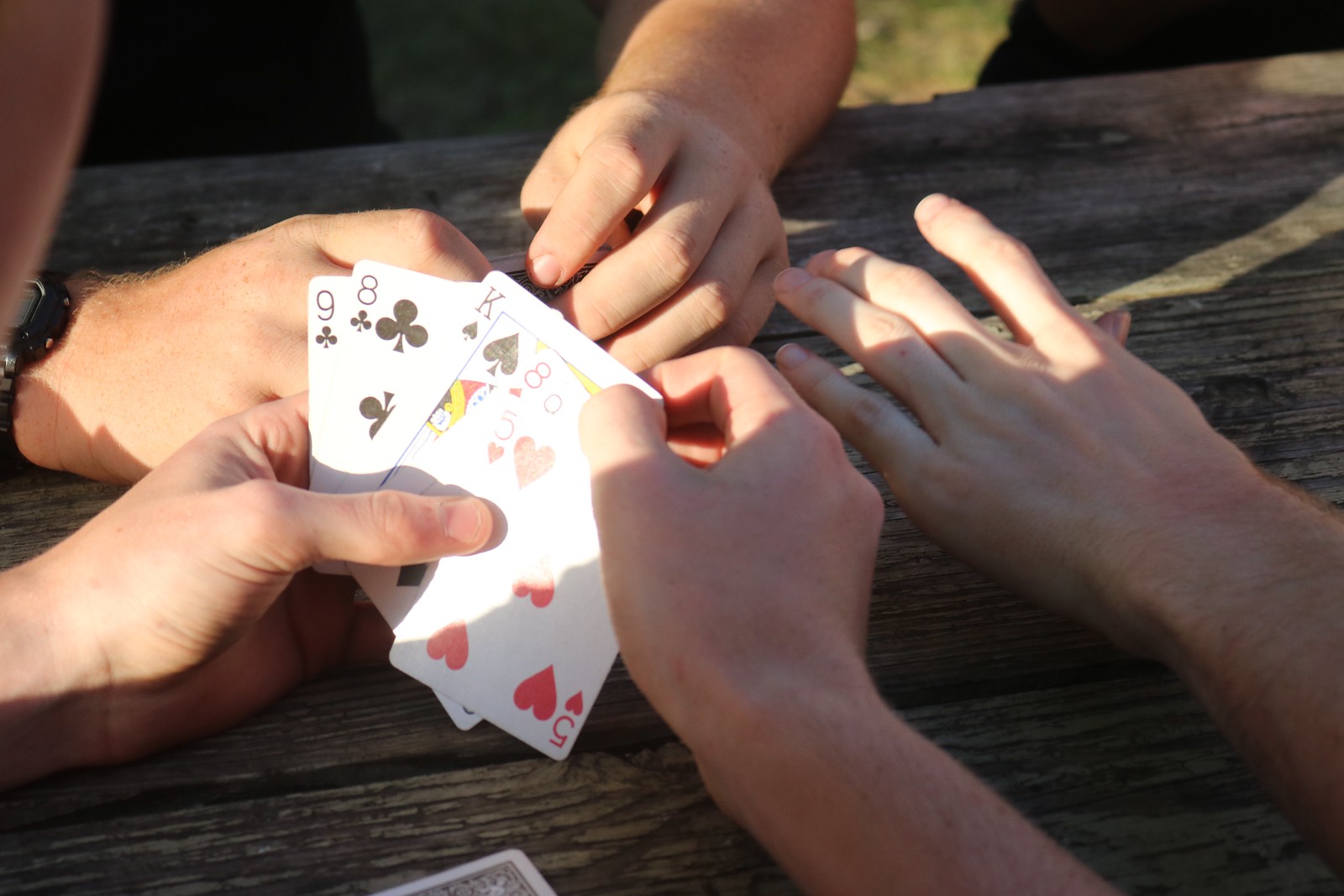In this photograph, a group of people are engaged in a casual card game at a weathered wooden table, likely a picnic table, showing signs of long exposure to the elements. The most prominent player, positioned closest to the viewer, displays their hand, revealing a nine of clubs, an eight of clubs, a king of spades, an eight of diamonds, and a five of hearts. Across the table, another player is visible, donning a large diving watch on their right wrist. This player holds their cards securely, preventing any view of the card faces or backs. A third participant’s left hand is partially seen, though their cards, if any, are not visible in the frame, suggesting they might be in the player’s right hand. The intimate scene captures the quiet focus and camaraderie of a classic card game.